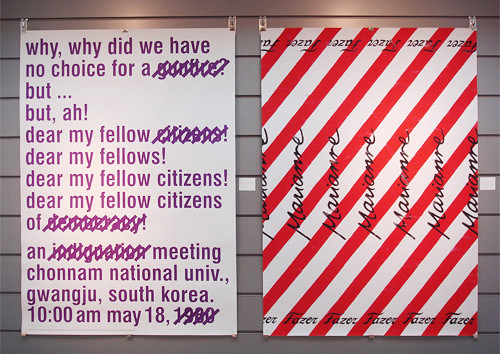The image depicts two posters pinned to a gray wall, each presenting distinct elements and text. The poster on the left is white with purple text and is clipped at the top. It begins by asking, "Why, why did we have no choice for a," followed by a word that is slashed through. Continuing, it reads, "But... but, ah, dear my fellow," with another word struck out, followed by "Dear my fellows, dear my fellow citizens of," and once more a word is struck out. Below, it announces a meeting at Chonan National University in Gwangju, South Korea, scheduled for 10 AM on May 18th, with the year '1999' partially struck out.

The poster on the right features a dynamic design of diagonal red and white stripes. It has black, flowing cursive text that vertically repeats the name "Marianne" across the middle. Additionally, the word "phaser" appears in the same cursive font both at the top and bottom of the poster, with the top instance being upside down. Together, these posters convey a mix of urgency and formality, with striking visual and textual presentations.